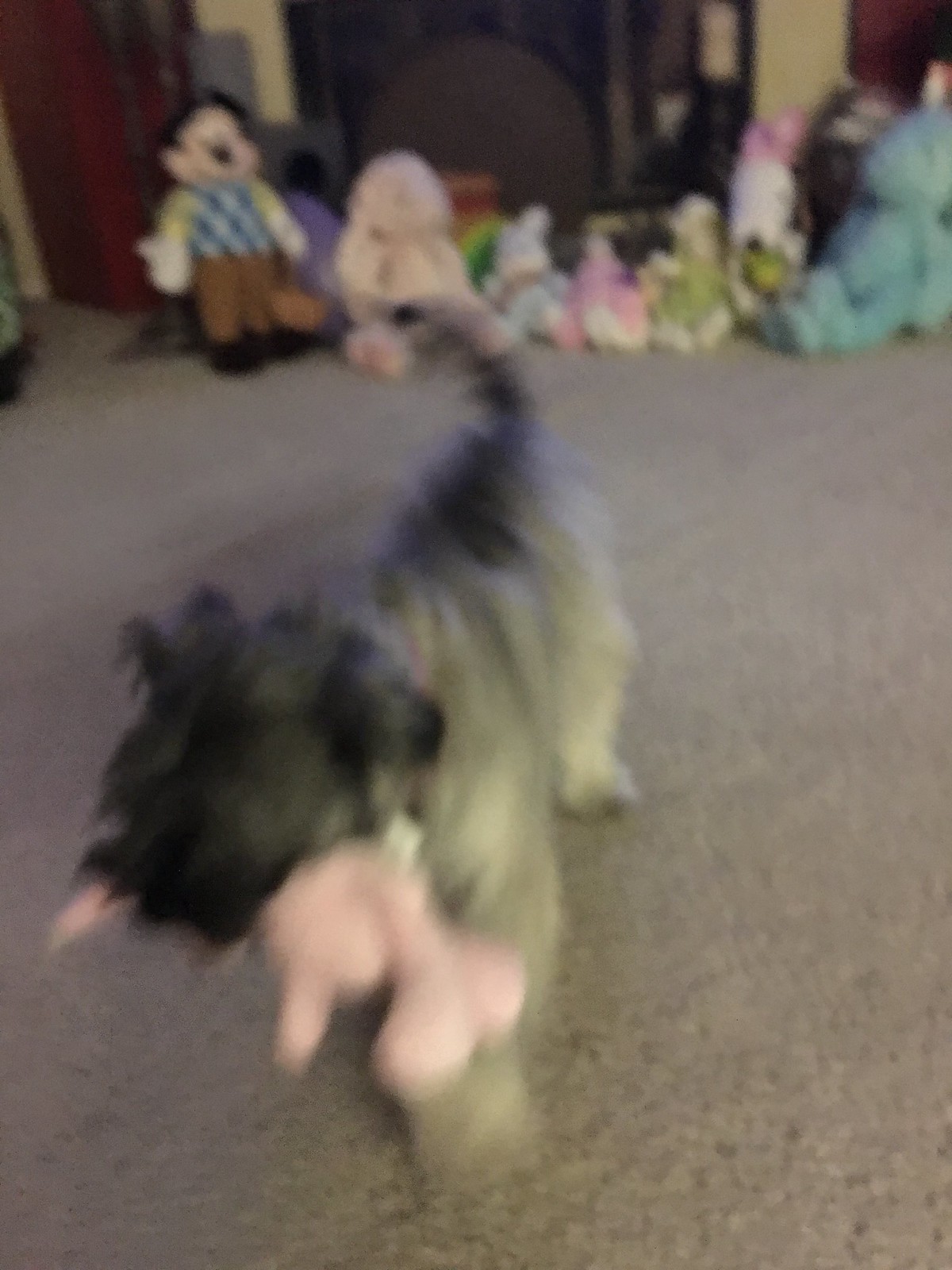In this blurry photograph, a small dog that resembles a Shih Tzu or terrier is captured holding a fluffy, light pink toy in its mouth. The dog features a predominantly dark black and gray face, with similar dark tones extending along the top of its back and tail. In contrast, its belly and legs are a lighter gray, verging on white. The dog is positioned facing towards the bottom left corner of the image, standing on a light tan carpet. The background reveals a collection of various stuffed animals arranged towards the top of the image, displaying a mix of colors and characters. Among them, a blue stuffed toy, a white one resembling Snoopy, a pink one, a bunny, and Mickey Mouse dressed in pants and a plaid shirt can be identified.